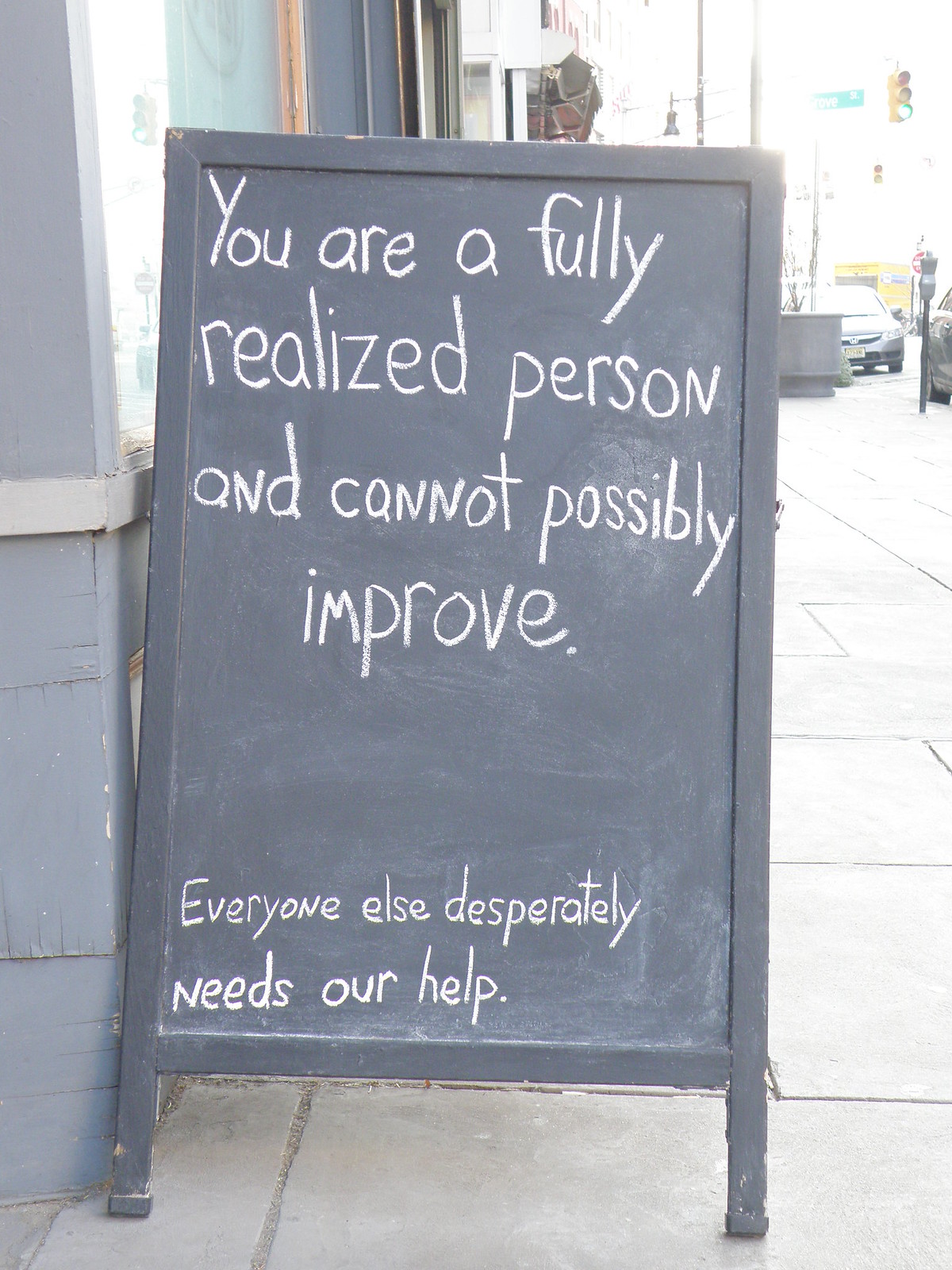The image portrays a collapsible black-framed chalkboard sign set on a cement sidewalk in broad daylight. The sign, situated against a blue-gray building on the left side, contains a message written in white chalk. The upper portion of the sign reads, "You are a fully realized person and cannot possibly improve," while the bottom half states in smaller text, "Everyone else desperately needs our help." In the background, there are cars, one parked beside a parking meter, and another either parked or moving along the street. The scene suggests a storefront setting with a typical urban street atmosphere.